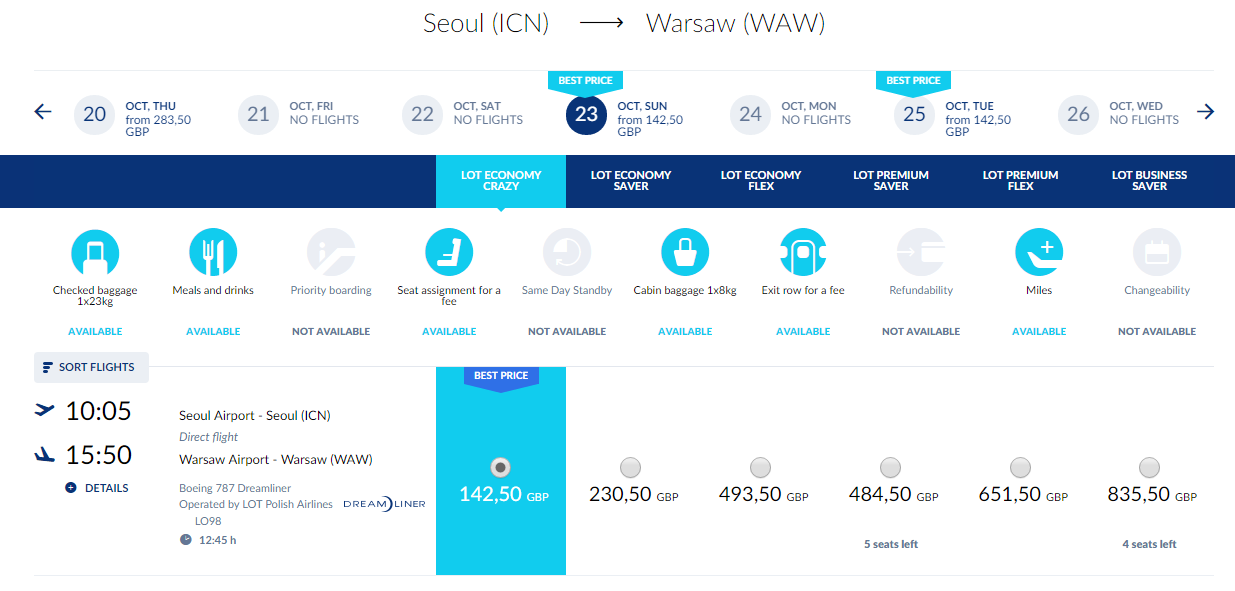**Detailed Caption:**

The image displays a flight information screen illustrating routes, dates, prices, and available services for flights from Seoul Incheon Airport (ICN) to Warsaw Chopin Airport (WAW). A forward arrow indicates the direction to Warsaw, while a back arrow shows a circular icon with the number 20. 

Below, the screen lists specific dates and prices: 
- **20th October, Thursday:** Prices starting from 283.50 GBP
- **21st October, Friday:** No flights available
- **22nd October, Saturday:** No flights available
- **23rd October, Sunday:** Highlighted in blue with a "Best Price" of 142.50 GBP
- **24th October, Monday:** No flights available
- **25th October, Tuesday:** Prices starting from 142.50 GBP and marked as "Best Price"
- **26th October, Wednesday:** No flights available

On the right, flight class options are detailed including: LOT Economy Crazy, LOT Economy Saver, LOT Economy Flex, LOT Premium Saver, LOT Premium Flex, and LOT Business Saver.

Additional services highlighted include checked baggage, meals and drinks, priority boarding, seat assignment, same-day standby, cabin baggage, exit row seating (for a fee), refundability, miles accrual, and changeability.